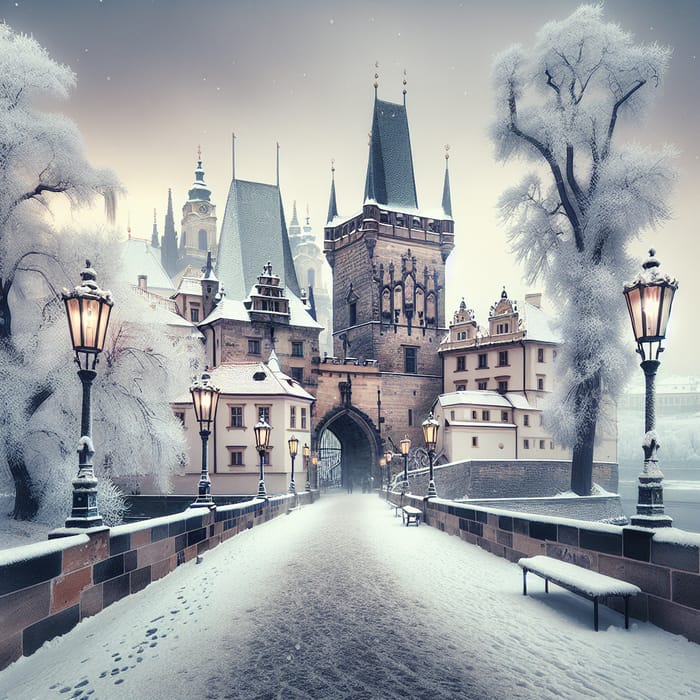This detailed 3D rendering or digital painting captures a serene, snowy scene of a bridge leading towards a city gate or castle courtyard amidst a tranquil night sky. The image is square in shape, approximately six inches both in height and width. The dark purple sky above is dotted with various white stars, gradually lightening to a cream color as it nears the city.

In the foreground, a snow-covered bridge extends toward the middle of the image, bordered by short brick railings made of large, multicolored stone blocks, three layers high. On the right side of the bridge, multiple four-legged benches without backs are lined up against the brick wall, all blanketed in snow. Streetlights or lanterns atop the stone barriers emit a warm, amber glow, illuminating the path forward. 

Footprints are visible in the snow on the left side of the bridge, hinting at minimal foot traffic, possibly from small animals. The pathway itself is relatively untouched by human presence, creating a sense of stillness and calm.

In the distance, tall buildings and an arched entryway or city gate loom grandly, indicative of a castle courtyard flanked by snow-covered trees with their branches devoid of leaves, instead adorned by a layer of white. The seamless blend of hues—from the grayscale elements of the buildings and pathway to the white and blue highlights in the snow— enhances the mystical, quiet ambiance of the scene.